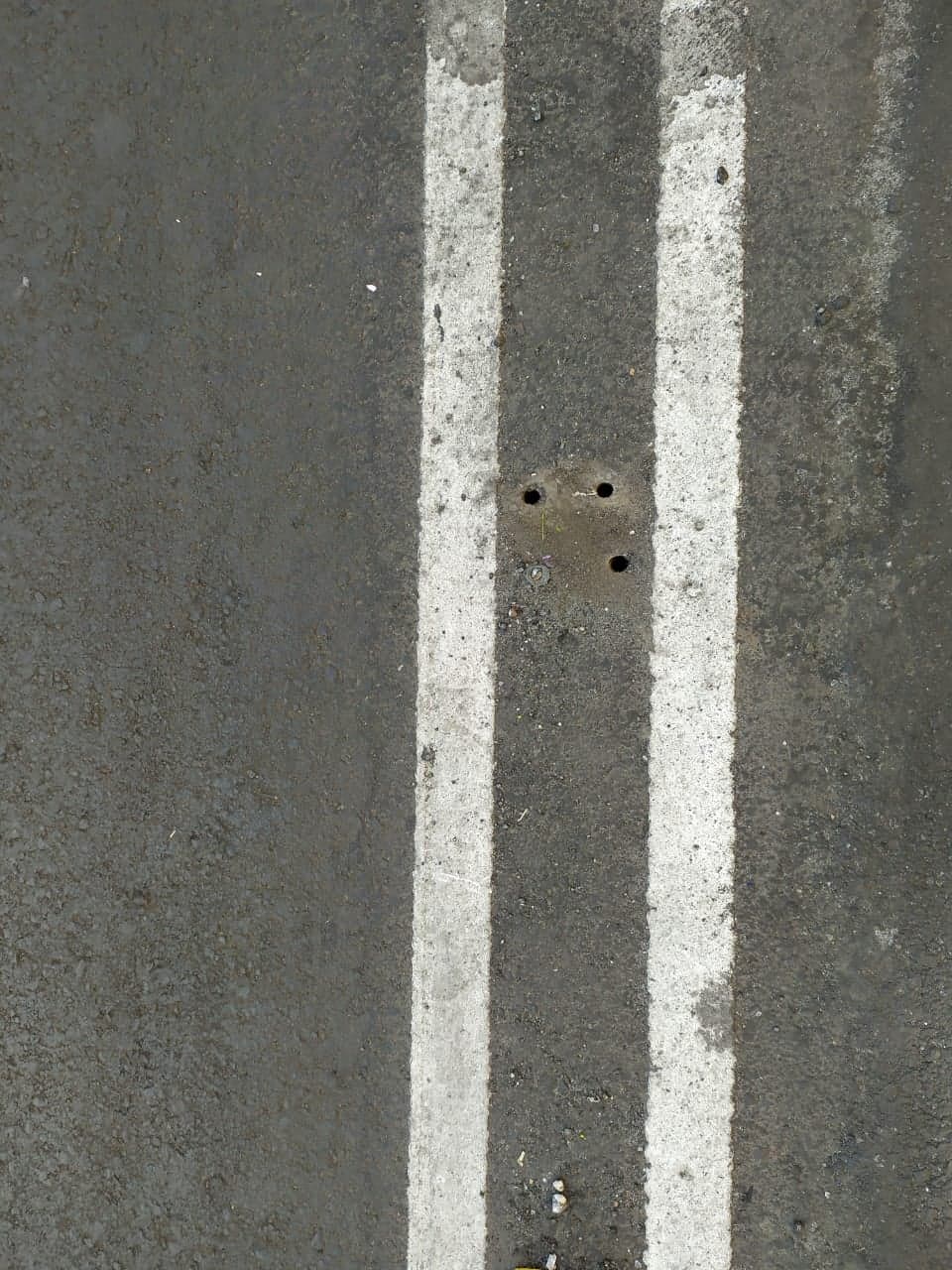This image depicts a close-up, aerial view of a gray street surface marked by two parallel white lines running vertically through the center. These lines are worn and chipped, revealing patches of gray asphalt beneath and creating an imperfect, weathered look. Littering the street are small rocks and debris, adding to the sense of wear and tear. Central to the image is a circular indention between the lines, with three small holes arranged in a triangular formation; a fourth, larger hole contains what appears to be a screw, suggesting the possibility of a missing cap. Inconsistencies in line alignment, as well as white speckles around the circular area, further contribute to the scene's textural complexity. No people or other objects are present, drawing attention solely to the peculiar details of the road surface.